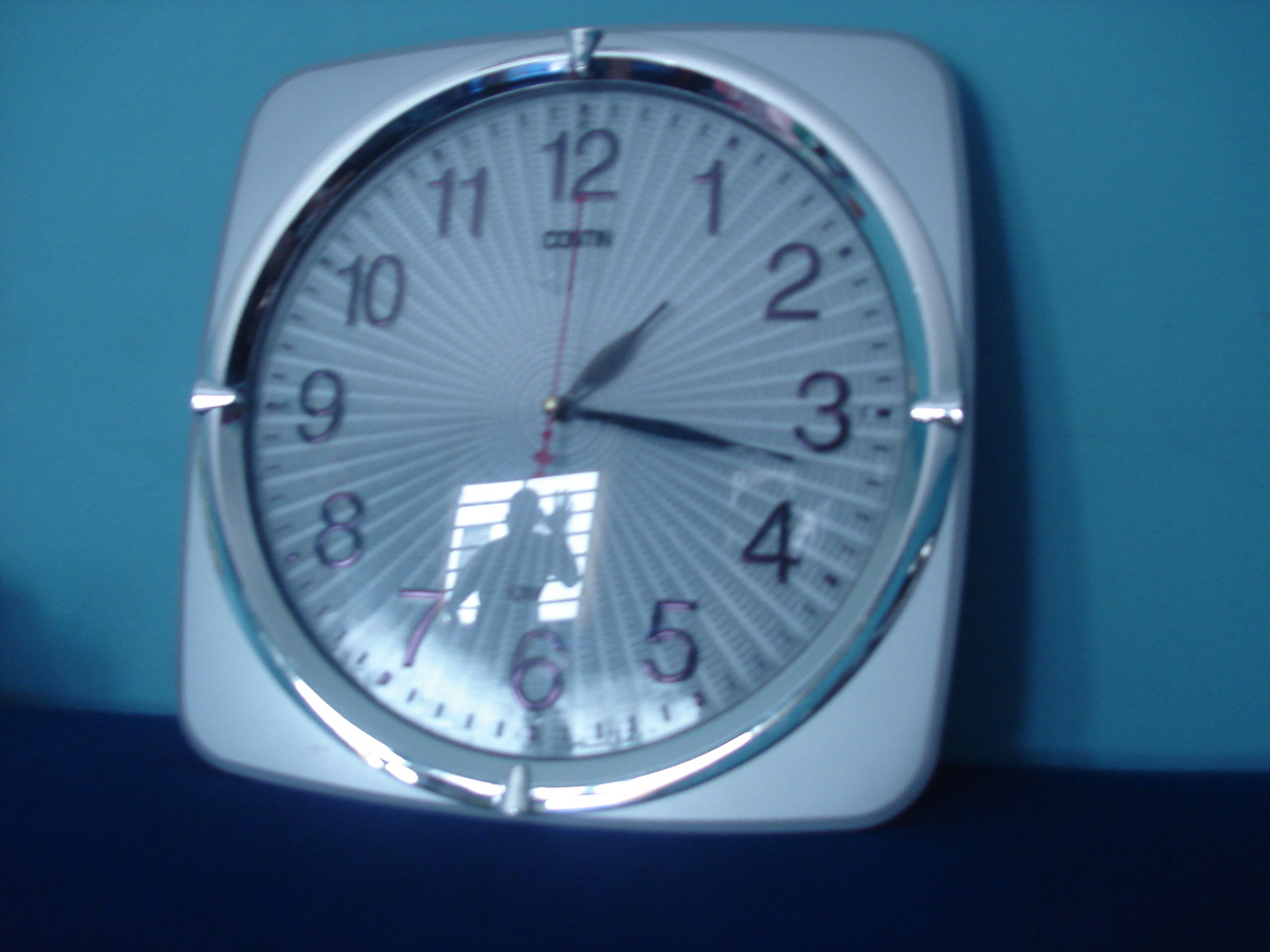This image features an old-school style clock with a bright silver outline and a distinctive radial design resembling fan-shaped pie slices, casting numerous shadows from the center. The round clock face is framed within a square aspect and displays numbers 1 through 12. The time indicates roughly 1:17, with the hour hand between 1 and 2, the minute hand between 3 and 4, and a prominent red second hand pointing straight up at 12. The silverish-blue clock is leaning against a blue background, either a wall or a couch, and supported by a darker blue shelf. Notably, there is a reflection on the clock face showing a window and a person's silhouette, likely that of the photographer, appearing ominously with a hand on the window between the 6 and 7 positions.